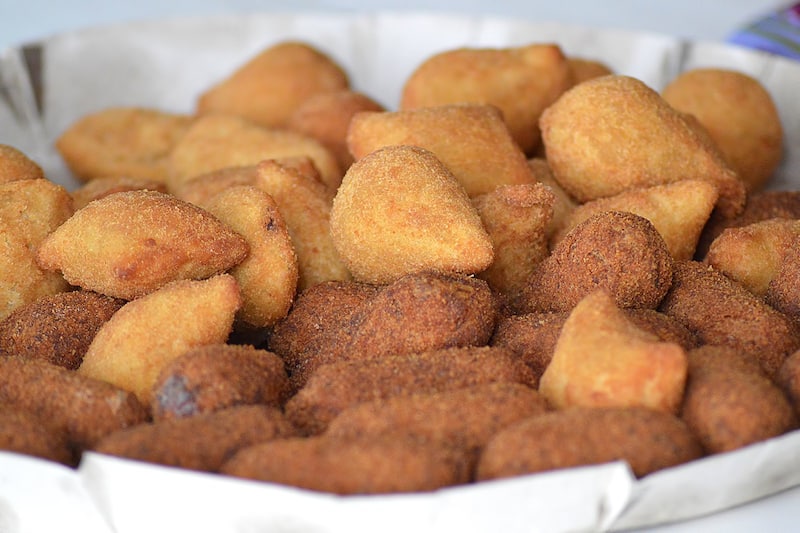The image captures a close-up view of approximately 30 to 40 bite-sized pieces of fried foods displayed in a white paper-like bowl. The items, which vary in shape from round to oblong and irregular, are coated in batter and differ in color. The majority at the top of the bowl are a golden yellow to light brown, suggesting they are lightly fried and could possibly be fried cauliflower or fritters, while the ones at the bottom are darker brown, indicating they were cooked longer. One piece is broken open, revealing a grayish interior. The background of the image is intentionally blurred but features a baby blue wall, and in the lower right corner, there is an indistinct blue item. Overall, the focus is on the texture and color contrast of the fried pieces, highlighting their crispiness and variety in doneness.